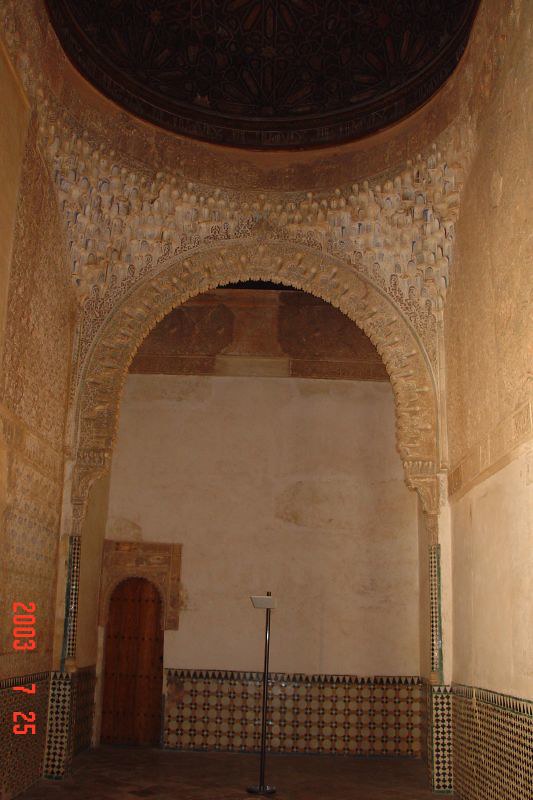This image depicts the interior of an ancient cathedral or religious structure, likely dating back many years. Dominating the scene is a large orange-hued archway that leads to a small room with a wooden door. To the left of the door, at the bottom corner, the date "2003-07-25" is visible, indicating when the photo was taken. The ceiling above the archway features a black, circular space adorned with intricate, though unclear, carvings and etchings, suggesting significant historical artistry. The surrounding walls are decorated with a mix of off-white, beige, and tan tiles, and the floor is a rich brown. Near the archway stands a vertical metal pole, possibly a microphone stand, adding a modern touch to the venerable setting.